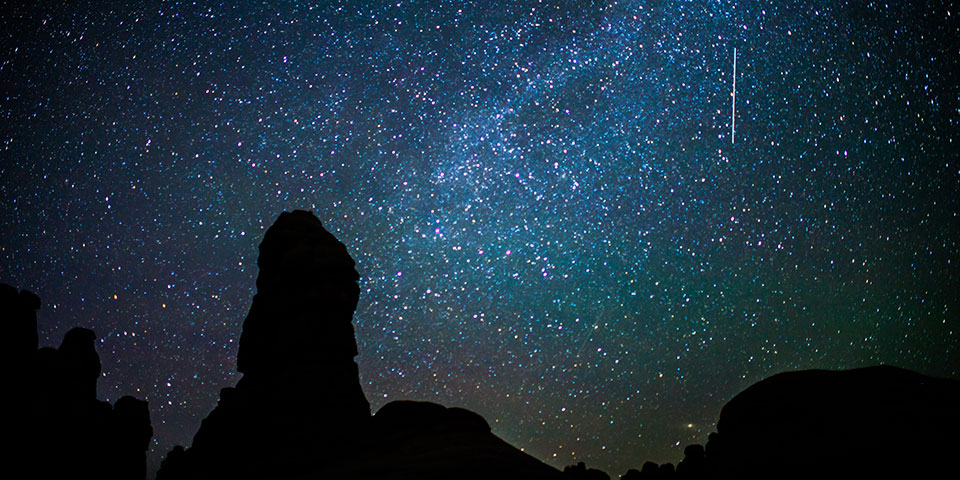This image depicts a mesmerizing night sky illuminated with a kaleidoscope of colors. The upper section of the sky exhibits a subtle bluish hue, transitioning into a rich green and teal gradient as it moves downward. Further down, a reddish tint emerges at the bottom, with a purplish hue visible to the left side of the picture. Scattered throughout the sky are countless specks of light in various colors such as purple, pink, orange, white, and blue, creating an enchanting starry nightscape. Particularly striking is a cluster of these dots situated in the middle of the sky. Toward the right side of this cluster, a distinct vertical white line cuts through the night. The foreground is dominated by the solid black silhouettes of rock formations, with the largest rock rising from the left side towards the middle of the image, and additional smaller formations stretching to the right. These shadowy rocks add depth and contrast to the vibrant celestial display above.